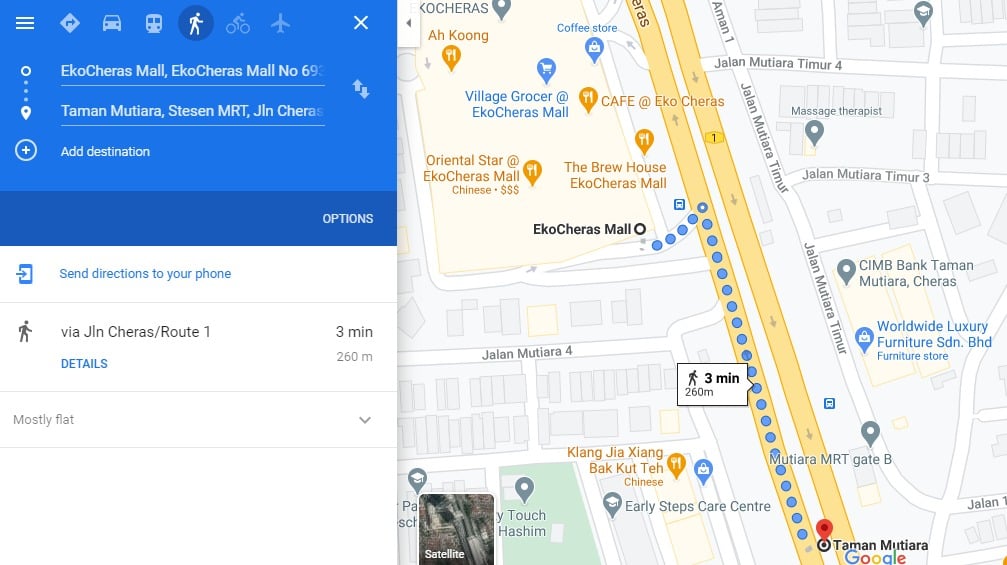The image is a screenshot of a navigational map interface. On the left side, there is a square section occupying about seven-eighths of the screen's width. The top portion of the square is a medium blue color, and it contains various transportation icons, including a car, a bus, a walking person, a bicycle, and an airplane. 

Below these icons, the text "Echocheris Mall" is displayed twice, followed by the number "693." The destination mentioned is "Taman Materia Stetson MRT, Gincheris."

At the bottom of this blue section, there is a darker blue banner with the word "Options" in white text aligned to the right. Beneath this blue area, on a white background, it reads "Send directions to your phone via J-L-N Cheras/Route 1." The estimated travel time is "3 minutes," and additional details include "260M" and "Mostly flat" in blue print.

To the right of this information, there is a map showcasing various streets, the specified destination, surrounding businesses, and notable points of interest like Echocheris Mall.